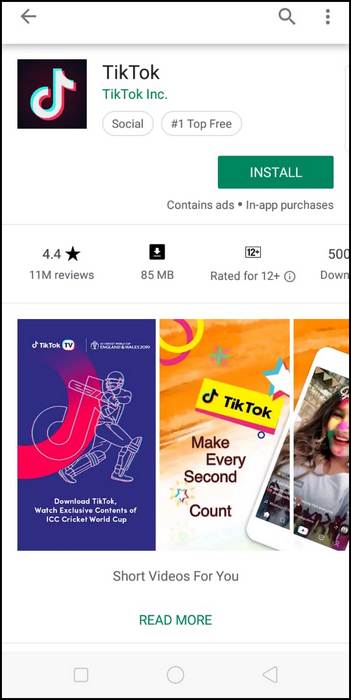The screenshot, set against a white background, prominently features the TikTok app listing. On the left side of the image, an arrow points toward a magnifying glass icon and three vertical dots. The text "TikTok" appears in black, while "TikTok Inc." is highlighted in green. An oval label displays "Social" alongside another oval labeled "No. 1 top free."

A green rectangle with the word "INSTALL" in white capital letters signifies the app’s installation option. Below this, the text indicates that the app contains ads and in-app purchases. The app has a rating of 4.4 stars from 11 million reviews. The download size is 85MB.

Additionally, there is a rectangle containing "Rated for 12+," displayed both textually and within a circle containing an eye icon. Below this section are three smaller rectangular images: 

1. The first rectangle, colored purple, depicts a dancing robot-like figure, accompanied by the text "TikTok TV" in white.
2. The second rectangle shows the phrase "Make Every Second Count" along with the bottom part of a phone.
3. The third rectangle completes the image of the phone, showing a girl smiling, suggesting she is either making a video or engaging in a chat.

This detailed visual layout aims to inform prospective users about the TikTok app's features, ratings, and installation details.